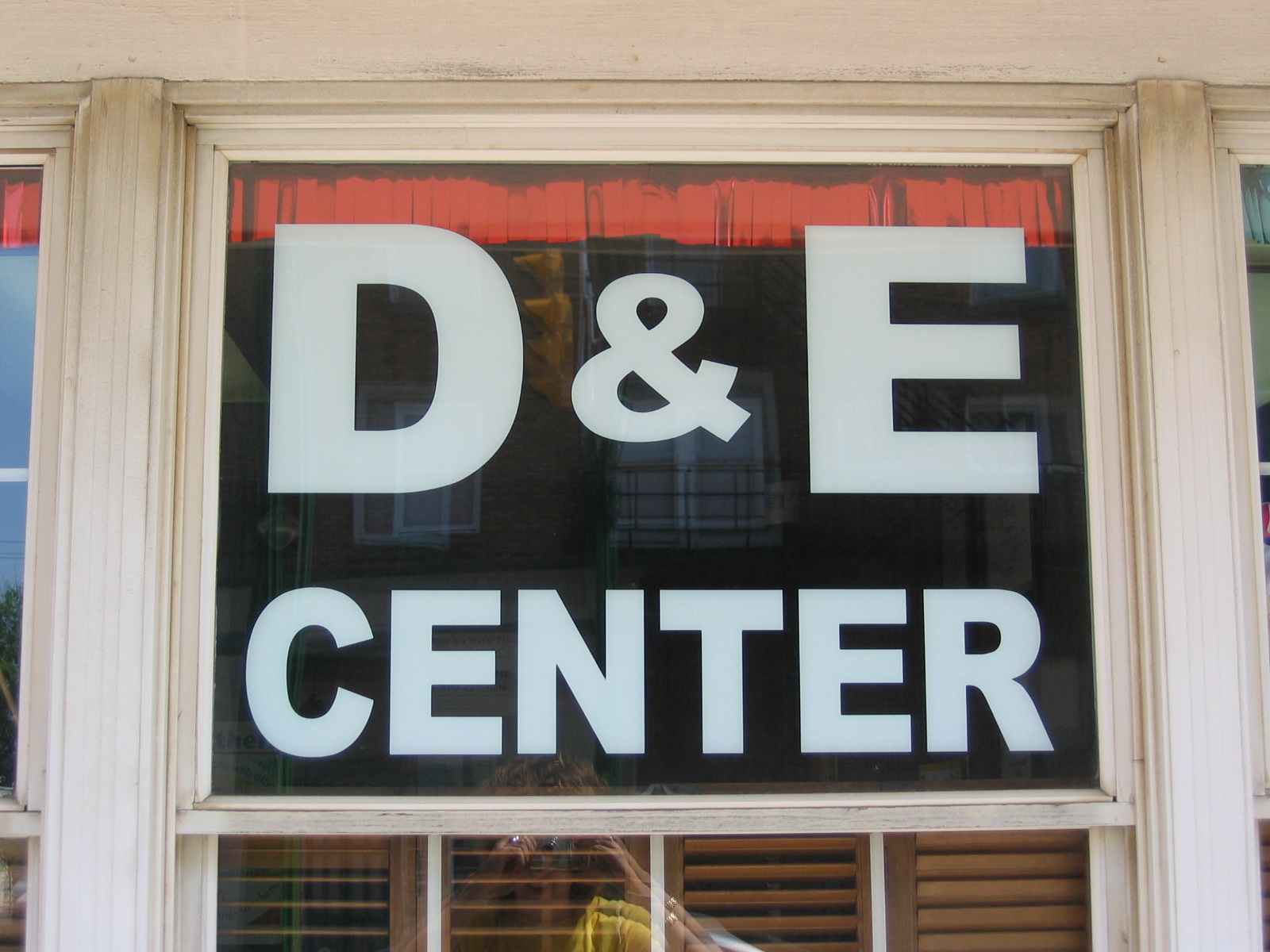The photograph features an old-school styled window with a white frame, slightly dirty, displaying the sign for a business called "D&E Center" in large white vinyl lettering. Instead of spelling "and," the sign uses the ampersand symbol (&). Below this main panel, the window contains brown wood shutters functioning as blinds. Red decor is faintly visible in the top section above the D&E lettering, adding a touch of color. On both the left and right sides of the image, slivers of neighboring windows are just noticeable. The reflection in the window captures the image of the photographer, identifiable by their yellow shirt, and hints at another building across the street. The external trim of the window is white and exhibits an old, traditional design.